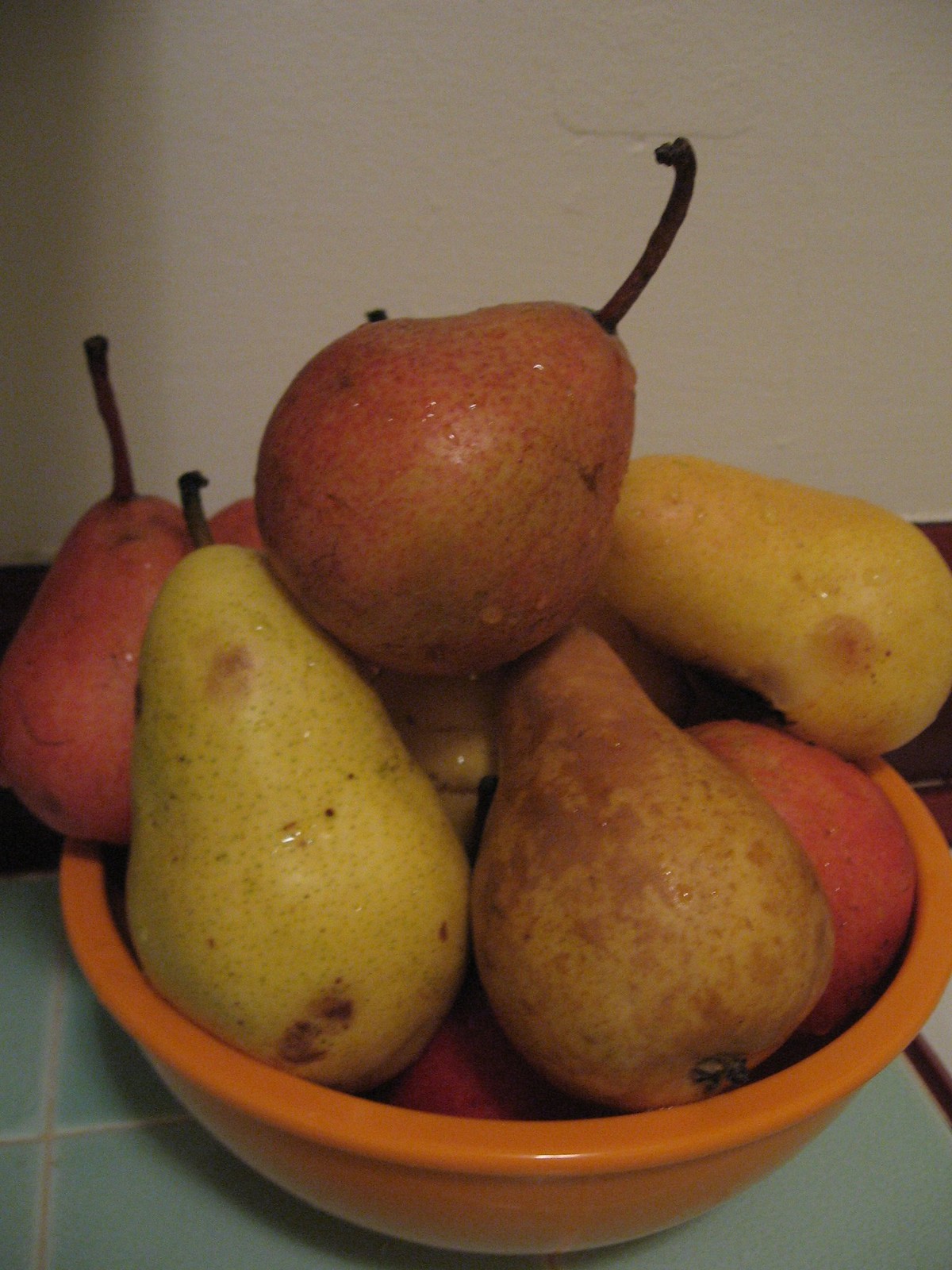The image is a very close-up, color photograph of a small, burnt-orange ceramic bowl overflowing with freshly washed fruit, set on an aqua-blue ceramic tile surface. The fruit, predominantly pears, is piled high above the rim of the bowl and extends outward. In the foreground, there are two pears: the one on the left is a pale green and yellow Danju pear with a couple of dark brown spots at the bottom and a lighter brown spot near the top. The adjacent pear is mostly brown with lighter greenish-yellow hues around the bottom. In the background and perched atop the foreground pears are several red, rounded fruits, likely apples or red pears, each with a prominent long brown stalk. The overall scene is situated in a kitchen with a white painted wall providing a plain backdrop, and the grout lines between the tiles form a noticeable light gray cross in the left-hand bottom corner of the image. The lighting is somewhat poor, emphasizing the natural textures and colors of the fruits and their slight bruises.